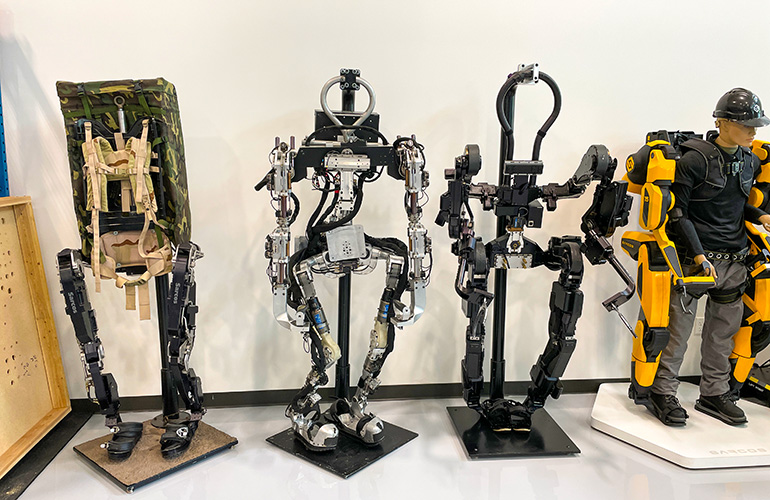The image depicts four exoskeletons in a room with a white background and black molding at the floor. Starting from the left, the first exoskeleton features a military-style camouflage backpack, black legs, and no visible arms, giving it a rugged appearance. The next exoskeleton is entirely silver, showcasing a sleek, robotic design with visible mechanisms that hint at how it would enable movement. Adjacent to it is another black exoskeleton, similar to the previous one but without distinctive features mentioned. Finally, on the far right, there is a yellow and black exoskeleton that resembles industrial models often used in warehouses. This exoskeleton is being displayed with a human-like doll inside, complete with a hard hat, illustrating its functionality and practical application. A wooden fence can be seen to the far left of the image, suggesting a potential outdoor or storage setting, and confirming the tall stature of these exoskeletons.